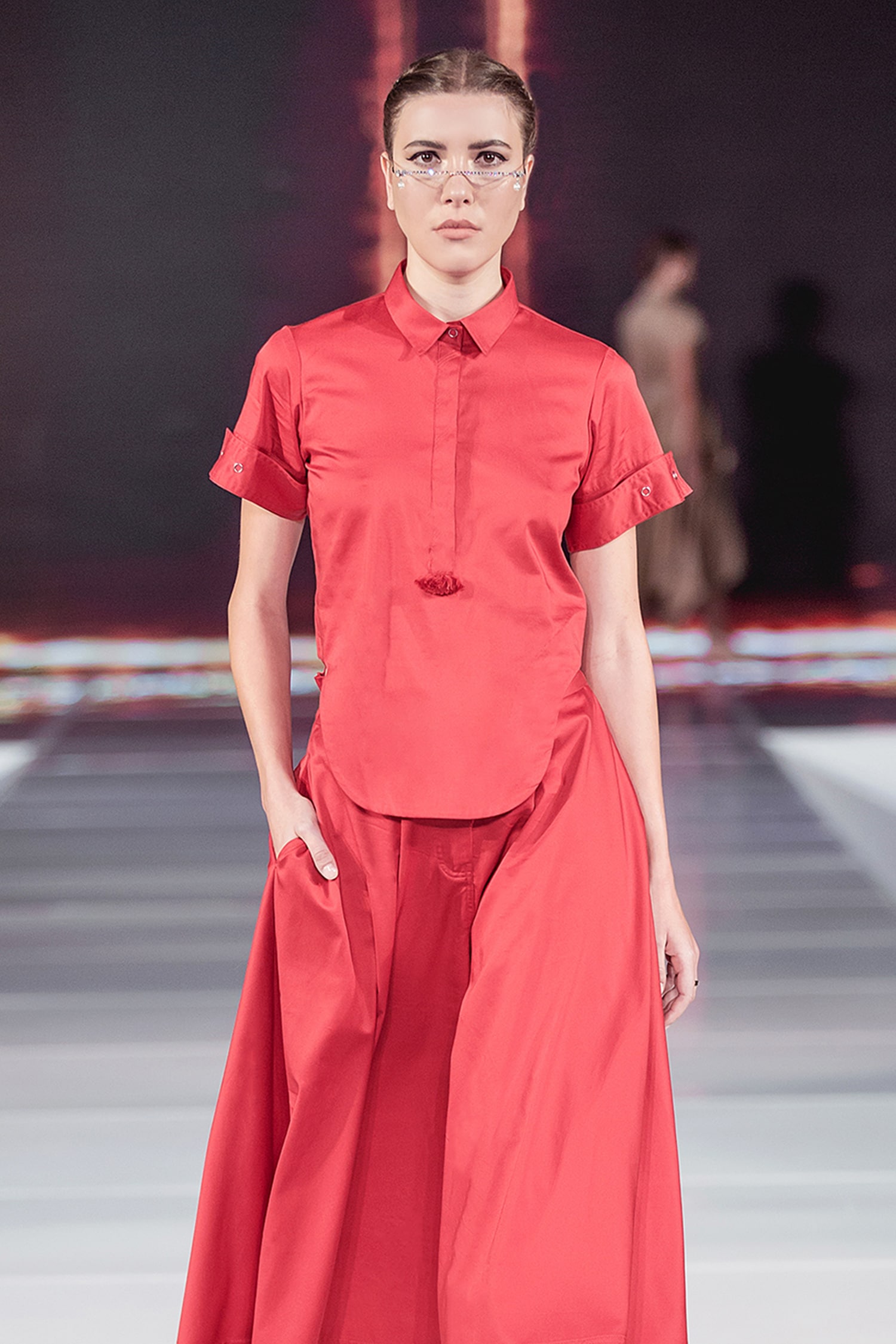This photograph captures a poised model striding confidently towards the camera on a runway, likely at a fashion show. The setting features a stage-like floor, black walls, and two striking red lines marking the entry and exit points behind her. The model epitomizes elegance in a cohesive red ensemble consisting of a short-sleeved blouse with a prominent collar and button-down front, effortlessly draped over a matching long skirt. Her right hand rests casually in her skirt pocket, while her left hand hangs naturally by her side. She has a natural makeup look with a pale face and subtle lipstick, and wears modern, contemporary glasses. Her brown hair is tightly slicked back, giving her a sleek and polished appearance. In the blurred background, another model can be seen walking, creating a dynamic and captivating composition.